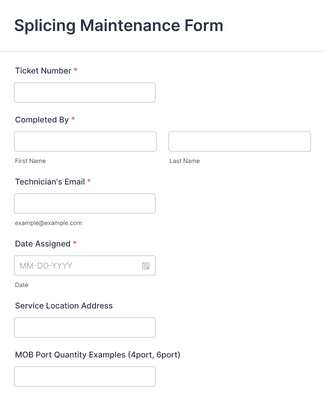The image showcases an online form designed for splicing maintenance. The form has a clean, white background, excluding the top inch, which is marked by a thin gray horizontal line stretching from the left to the right of the page. Above the line, in bold black letters, is the title "Splicing Maintenance Form," with each initial letter capitalized. 

Directly beneath the title is the label "Ticket Number," which appears in smaller black letters and is followed by a red asterisk, indicating a required field. Corresponding to this label, there is a rectangle input box extending about halfway across the page. Below this section, the label "Completed By" is displayed, again with a red asterisk beside it. Next to it is another rectangle input box of the same width. 

Further down, the form splits into two parts for "First Name" and "Last Name." The "First Name" field is enclosed in a rectangle stretching halfway across the page, while the "Last Name" field, located to its right, extends from the middle of the page to the right edge.

Proceeding to the next section, the label "Technician's Email," marked with a red asterisk, is followed by a rectangle input box going halfway across the page. An example email "example@example.com" is provided beneath this input box for reference.

Next, the form features the "Date" field, indicated by a red asterisk. This section has an input box extending halfway across the page, with a placeholder text "mm-dd-yyyy" and a small calendar icon on the right side within the box.

Below the "Date" field, the label "Service Location Address" precedes another rectangle input box, also stretching halfway across the page. At the bottom of the form, there is a unique section labeled "M-O-B P-O-R-T Q (Examples: '4-Port, 6-Port')" in capital letters. This field is accompanied by an input box, matching the width of previous ones, located directly beneath the label.